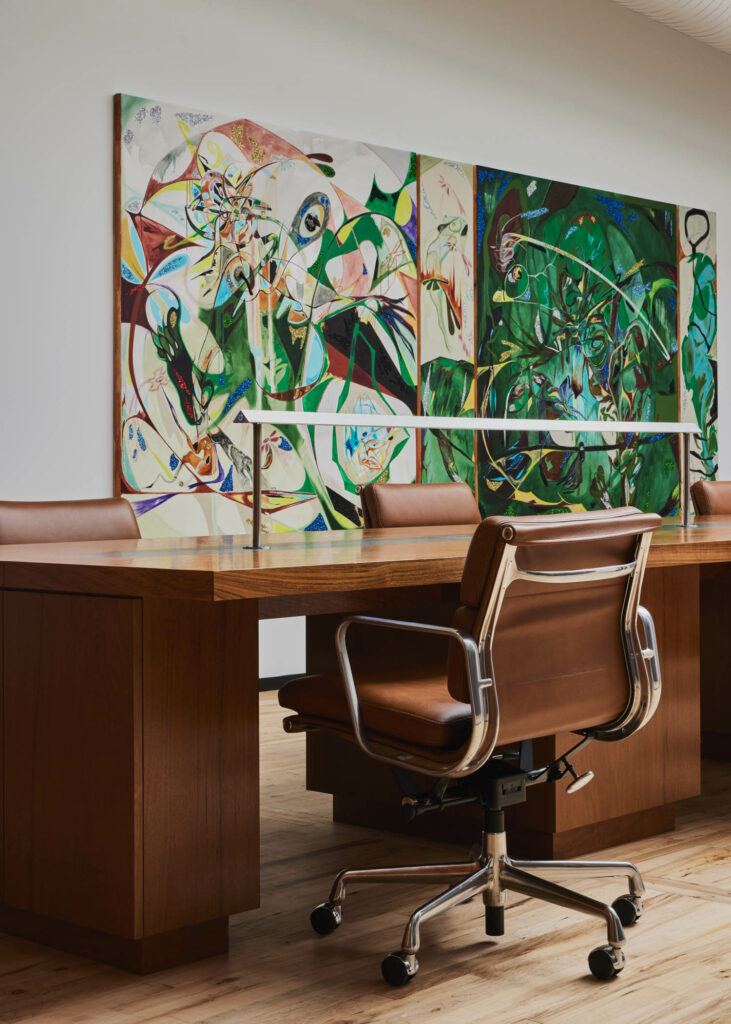This image depicts a possible office or boardroom setting featuring a dark, wooden table that extends beyond the right edge of the photograph. Along the table are brown leather office chairs with chrome metal frames and wheels, three of which are fully visible with part of a fourth chair on the right. The tabletop is very shiny, with a long, abstract lamp positioned in the middle, standing about a foot and a half high. The wooden floor complements the table's dark finish. The white wall behind the table is adorned with several large, vibrant abstract artworks. These artworks introduce a burst of colors including green, red, orange, purple, yellow, and blue, with one piece having a predominantly white background and another mostly green and blue. The dynamic art adds a slightly retro and Scandinavian feel to the room.